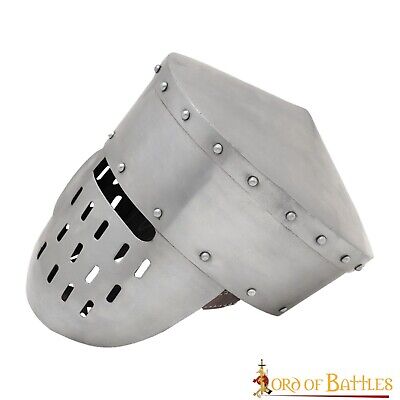This side-view photograph captures a medieval helmet and face mask made of hammered silver metal. The helmet features a pointed top with rivets running along both the upper and lower edges. The face mask, designed in a hockey mask style, presents a multitude of holes cut out from the metal, likely for breathing, alongside a distinct slit for the eyes. The mask gives the impression of being secured to the face by the attached metal helmet. At the bottom right of the image, there is a "Lord of Battles" logo, inscribed in an ancient, medieval font on a white background. The "L" in "Lord" is artistically designed to resemble a sword.